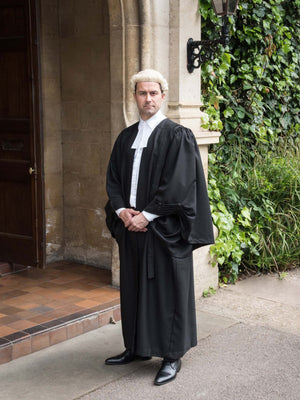This vertical photograph captures a stern-faced man dressed as a judge standing outside in front of an elegant stone building. The man, wearing a black judicial robe over a white shirt and cravat, dons a traditional white curly wig typical of English and Canadian judiciary attire. His black pointed shoes contrast sharply with his white ensemble, and he stands with his hands folded together in front. To his left, the building made of beige to light gray stones features a prominent pillar at the center adorned with an ornate black wrought iron lamp post. An open dark brown wooden door with a gold handle is situated to the left, preceded by a step of reddish-brown tiles. Beneath the step, there are gray concrete slabs extending towards the right. Above and behind the pillar, lush green ivy climbs the stone wall, interspersed with thick green grass. The entire scene is framed with a slightly blurred background, emphasizing the man’s solemn expression and traditional attire.